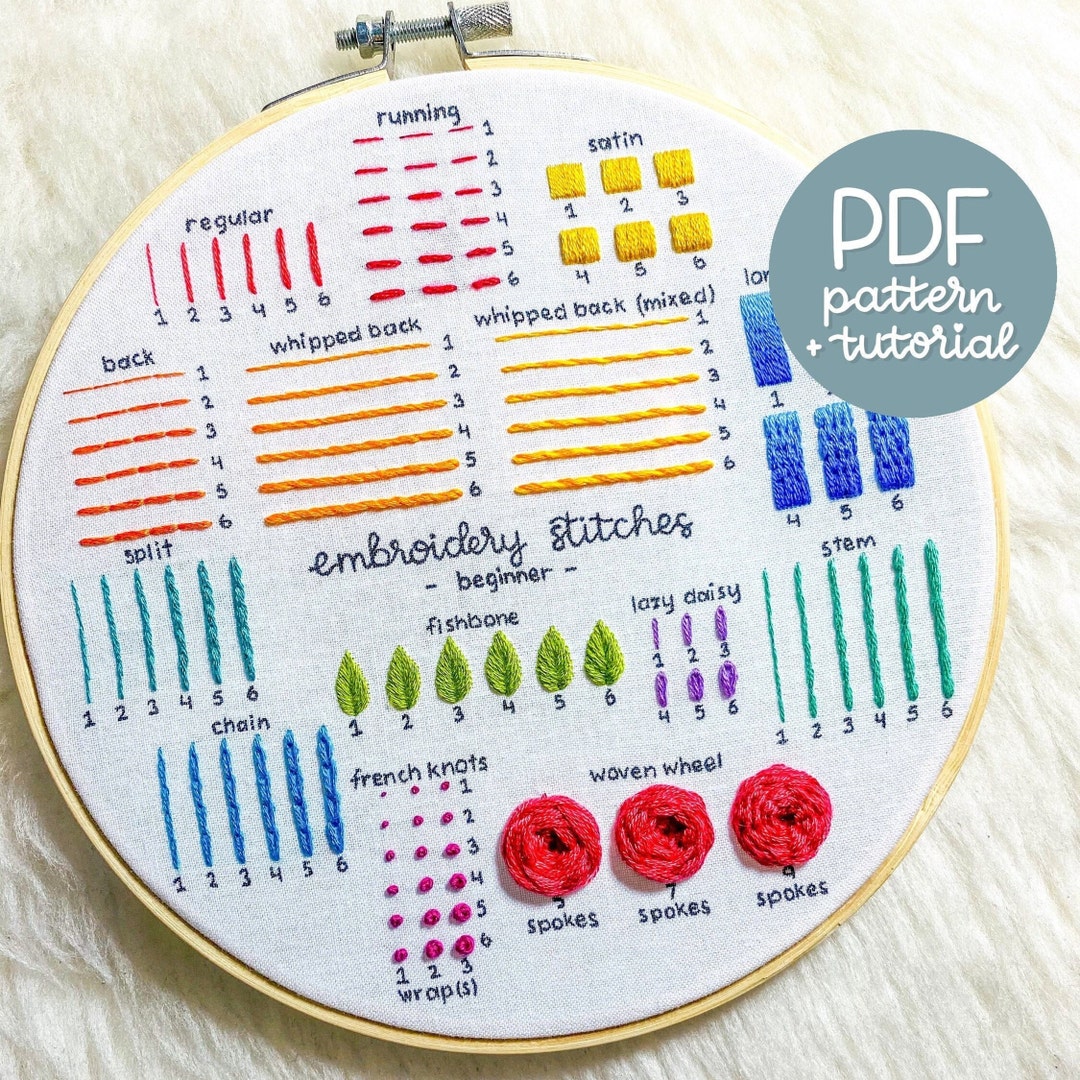The image shows a round embroidery hoop, featuring white fabric stretched taut within the hoop, set against a textured, white fur background. In the top right corner, a cyan circle with white text reads "PDF pattern and tutorial." The central inscription on the fabric states "Embroidery Stitches Beginner." The fabric is adorned with various examples of stitch techniques in a spectrum of colors, including red, yellow, orange, blue, green, and purple. At the top, the stitches demonstrated include Regular, Running, and Satin, shown in red and yellow. Below these, other stitches are labeled, such as Back, Whipped Back, Whipped Back Mix, and a partially obscured label. Further down, more types of stitches are illustrated, including Split, Stem, Lazy Daisy, Fishbone, Chain, French Knots, and Woven Wheel. Each stitch type employs different colored threads to clearly differentiate the designs.